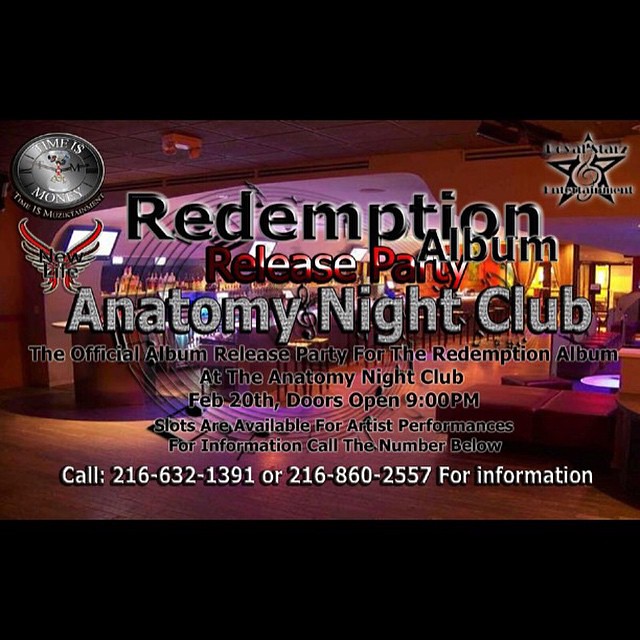The image is a vibrant advertisement for the Redemption Album Release Party at Anatomy Nightclub on February 20th. Dominated by hues of red, purple, orange, and burgundy, the backdrop reveals glimpses of the nightclub, including its bar, booths, and tables, with bright yellow lighting creating a nighttime club atmosphere. Superimposed text announces the event details: "Doors open at 9 p.m.," and "slots are available for artist performances." Contact information for more details is provided with two 216 area code numbers in white font. In the upper left corner, a silver coin-like logo reads "Time is Money" and "Management," while the upper right corner features a star logo. An emblem with red and white wings is also visible, enhancing the dynamic and promotional nature of the advertisement.